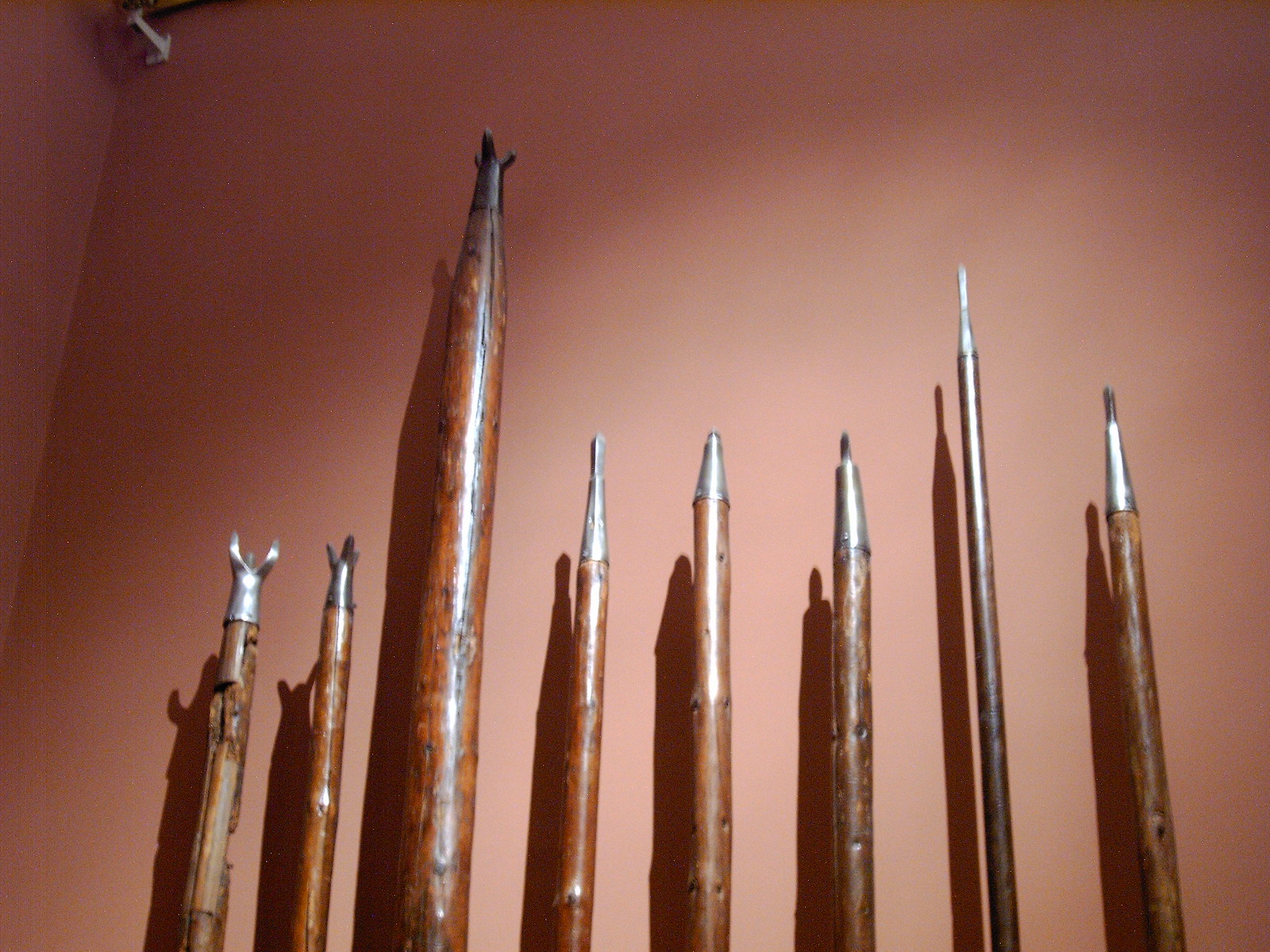The image is a slightly out-of-focus, indoor color photograph capturing a close-up view of eight handmade wooden lances with metal tips, displayed against a pinkish to reddish-brown wall corner. The lances, appearing authentic and possibly antique, are arranged vertically, with varying heights and diameters. The first two lances on the left are short and equipped with three-pronged metal claw tips. The third lance is significantly taller and thicker than the others, featuring a three-pronged metal tip. The middle three lances are slimmer, with pointed metal tips, one of which is particularly narrow and straight. The seventh lance resembles the middle ones but is slightly stouter and taller. The last lance also has a sharp pointed tip. Shadows from the lances are cast on the wall due to a light source coming from the upper right. In the upper left corner of the image, a white fixture, possibly a bracket or security device, is visible. The overall tone of the image suggests the lances might be artifacts from the turn of the century if not older.